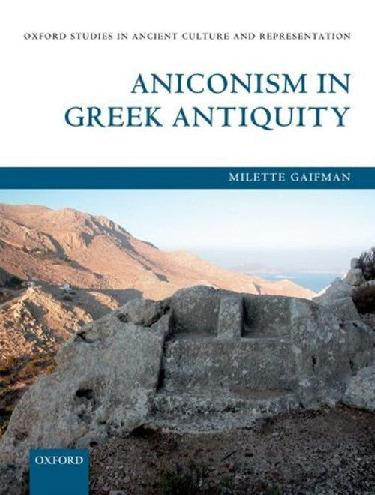The front cover of the textbook, titled "Oxford Studies in Ancient Culture and Representation," features an image set against a white background. The title is prominently displayed at the top in black letters. Below this, in blue letters, is the book’s specific title, "Aniconism in Greek Antiquity." A horizontal blue rectangle spans the page underneath, with the author's name, Millet Giffman, written in white letters. Dominating the lower portion of the cover is an evocative outdoor landscape depicting ancient ruins. This scene includes a dry, arid environment with rocky formations in varying shades of brown and gray, situated along a mountaintop under a blue sky. A notable feature is a body of water on the right-hand side, contrasting with the rock formations extending towards the middle. At the bottom-left corner, a blue square with the word "Oxford" in white letters is featured, adding a distinct touch to the cover design.